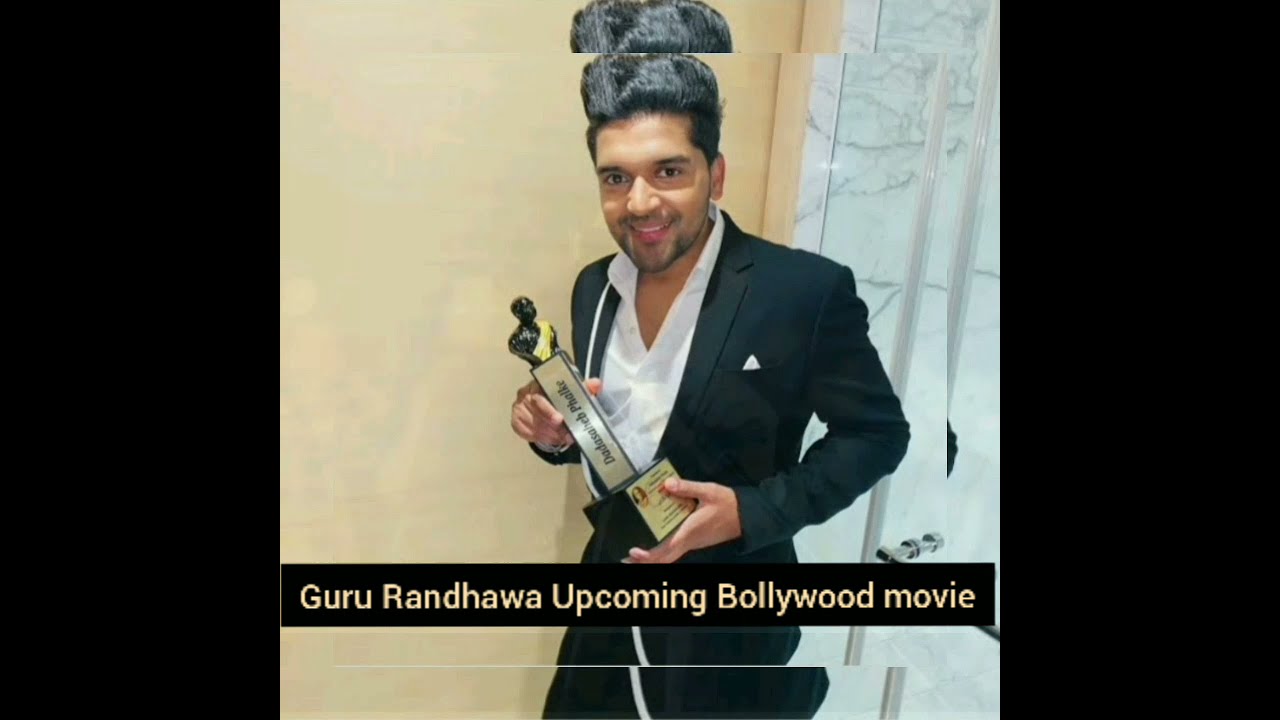This is a detailed photograph of a South Asian man, presumably Indian, with light caramel-colored skin and shiny black hair, posing indoors. He is centered in the image, smiling and looking directly at the camera. Dressed in a black coat and a white shirt with the upper button undone, the man's appearance is professional and polished. He holds an elaborate trophy in his hands, which is black, silver, and golden in color, featuring a statue on top. 

The backdrop exhibits a light brown wall to the left and some curtains on the right. Additionally, there is a piece of marbled slab with grey veins and a silver door handle visible on the right. At the bottom of the image, a black bar contains text in a beige font, reading "Guru Randhawa, Upcoming Bollywood Movie." The setting suggests this is a professional photo taken at an awards ceremony or a similar event, with vertical black strips framing the image on both sides.

This composition includes a variety of colors such as black, white, silver, gold, tan, and light brown, contributing to the sophisticated atmosphere of the scene.